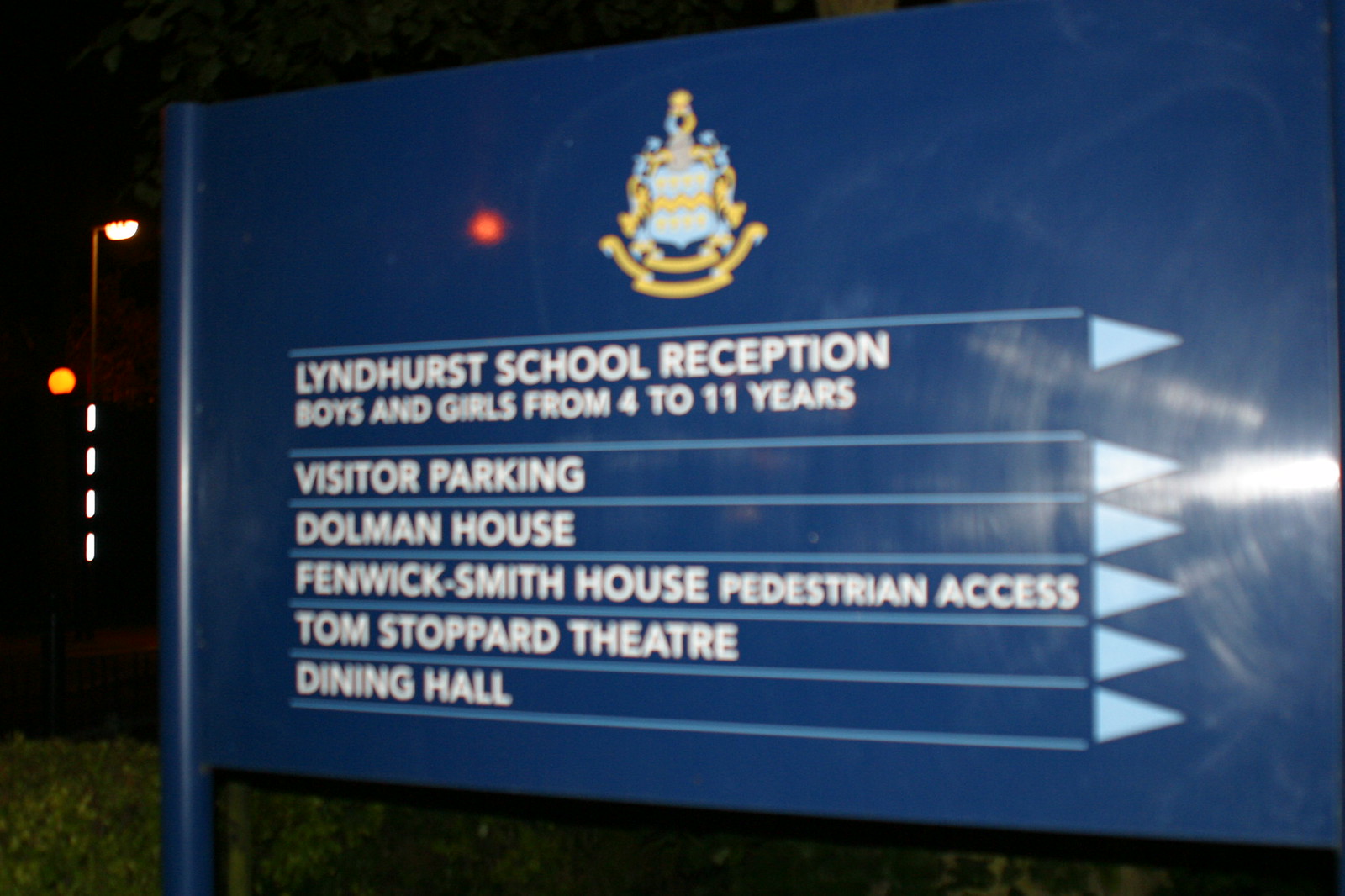The image captures a nighttime scene with a dark background, illuminated by distant street lights and a red light reflecting on a prominent metal sign. The sign, framed against grass-covered ground, is primarily a dark blue color with white lettering and accents. Crowning the sign is a yellow and blue emblem. The detailed writing on the sign reads: "Lindhurst School Reception," followed by "Boys and Girls from 4 to 11 years," "Visitor Parking," "Dolman House," "Fenwick Smith House," "Pedestrian Access," "Tom Stoppard Theater," and "Dining Hall." Each line of text is underlined with a light blue line that extends to a blue triangle, pointing right.